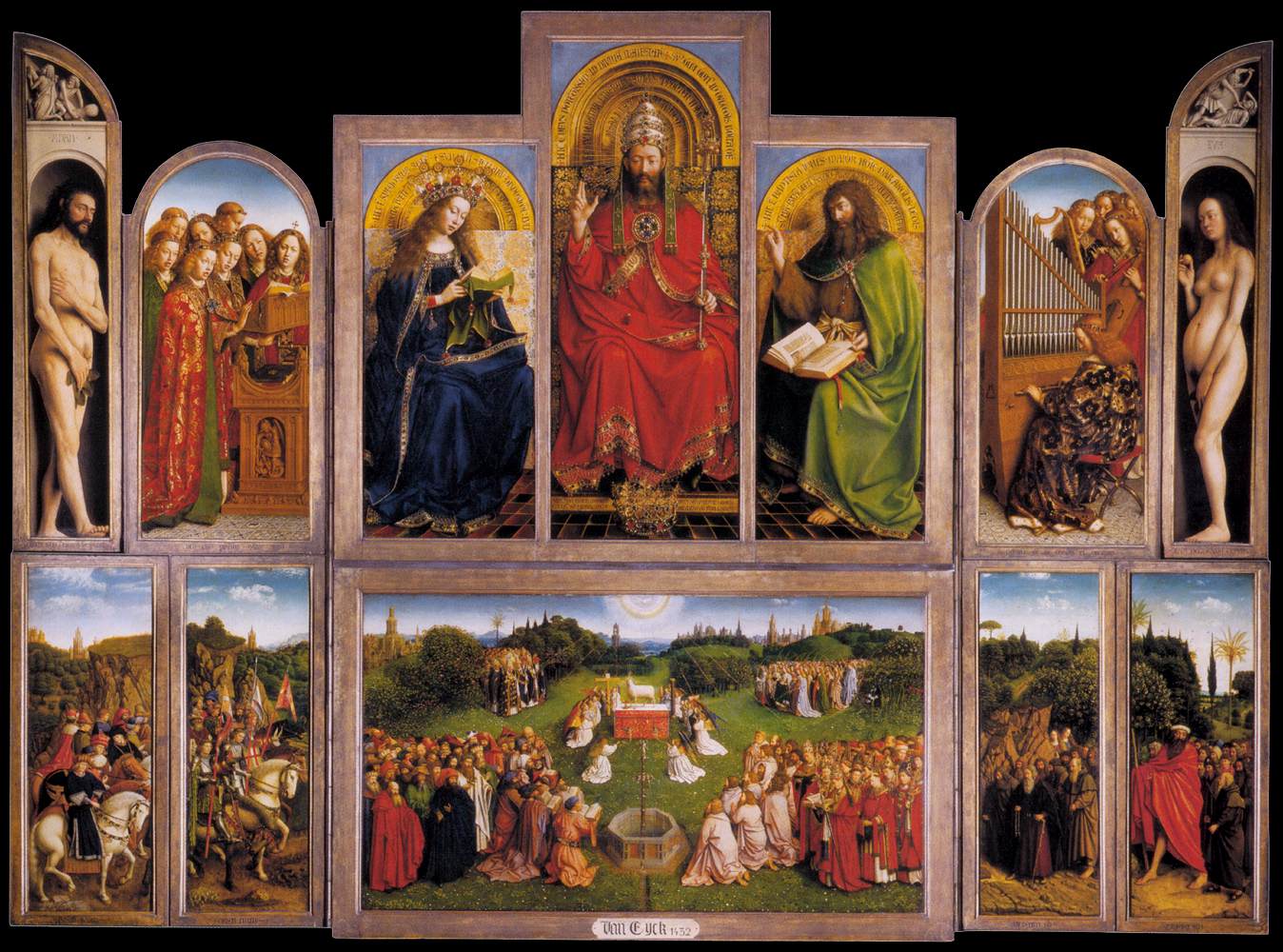The image showcases a series of old religious paintings arranged in the triptych style with central and hinged side panels. At the top, the main triptych features three distinct panels: the left panel displays a naked man covering his groin with an olive leaf, likely Adam; the right panel shows a naked woman, possibly pregnant, covering herself with a similar leaf, presumably Eve. The central panel features a throne with a figure wearing a tiered helmet or crown, flanked by two robed individuals. Below this, another triptych depicts a vibrant garden scene where people are gathered around a well or fountain, suggesting a worship ceremony centered around a lamb on a pedestal. The left side of this bottom triptych shows people on horseback, dressed in royal regalia resembling knights, while the right side presents more figures walking along a dirt path. The paintings, housed in rectangular wooden frames—with some frames arching at the top—display a blend of indoor biblical scenes with outdoor garden vistas, emphasizing intricate details and a rich narrative of religious iconography.